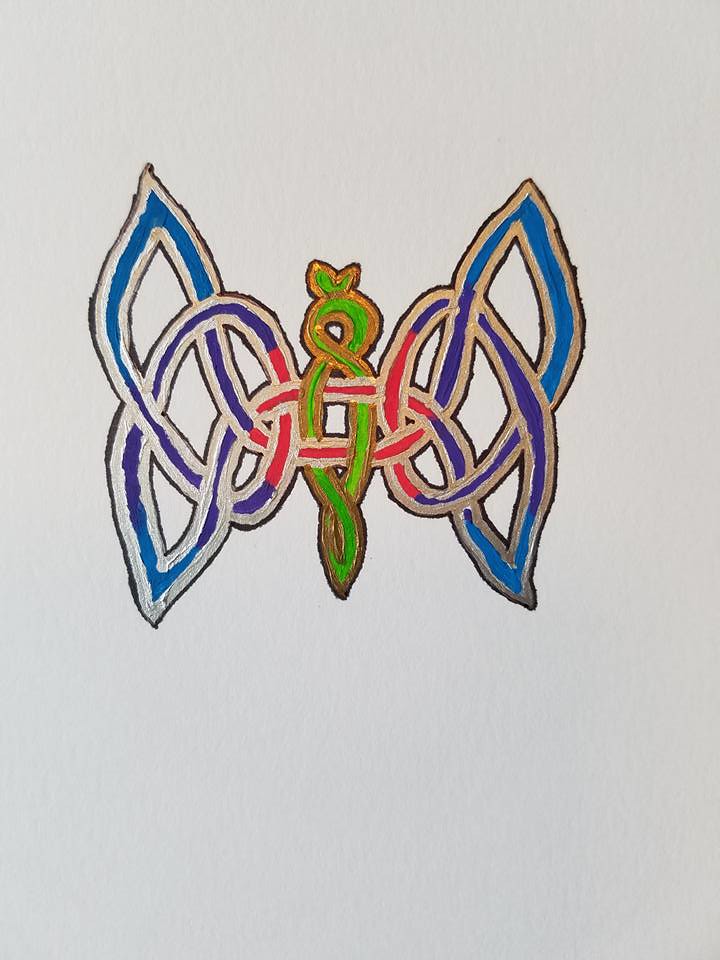The artwork features a detailed, hand-drawn butterfly with a paint-marker aesthetic, giving it a glossy, slightly clumpy texture due to the buildup of the paint. Set against a light gray background, the butterfly’s design includes an intricate, symmetrical pattern suggesting a tapestry or Persian rug motif. 

At the center of the butterfly is a twisted looped knot that looks like its body, bordered in gold with a green interior. This central body extends to a circular shape at the top, resembling a head with small antennae. From the body, two wings unfurl, starting with a deep pink color near the center, transitioning through dark blue, and ending in sky blue at the tips. Each wing is outlined in silver and a darker gray, enhancing the decorative aesthetic.

The wings themselves are split into four parts, with two sections on each side. These forms loop, weave, and interconnect like a pretzel or silly straw, imbuing the butterfly with a sense of movement and complexity. Red ovals with silver outlines adorn the design, standing out from the interlacing lines, which are meticulously bordered in black for a striking contrast.